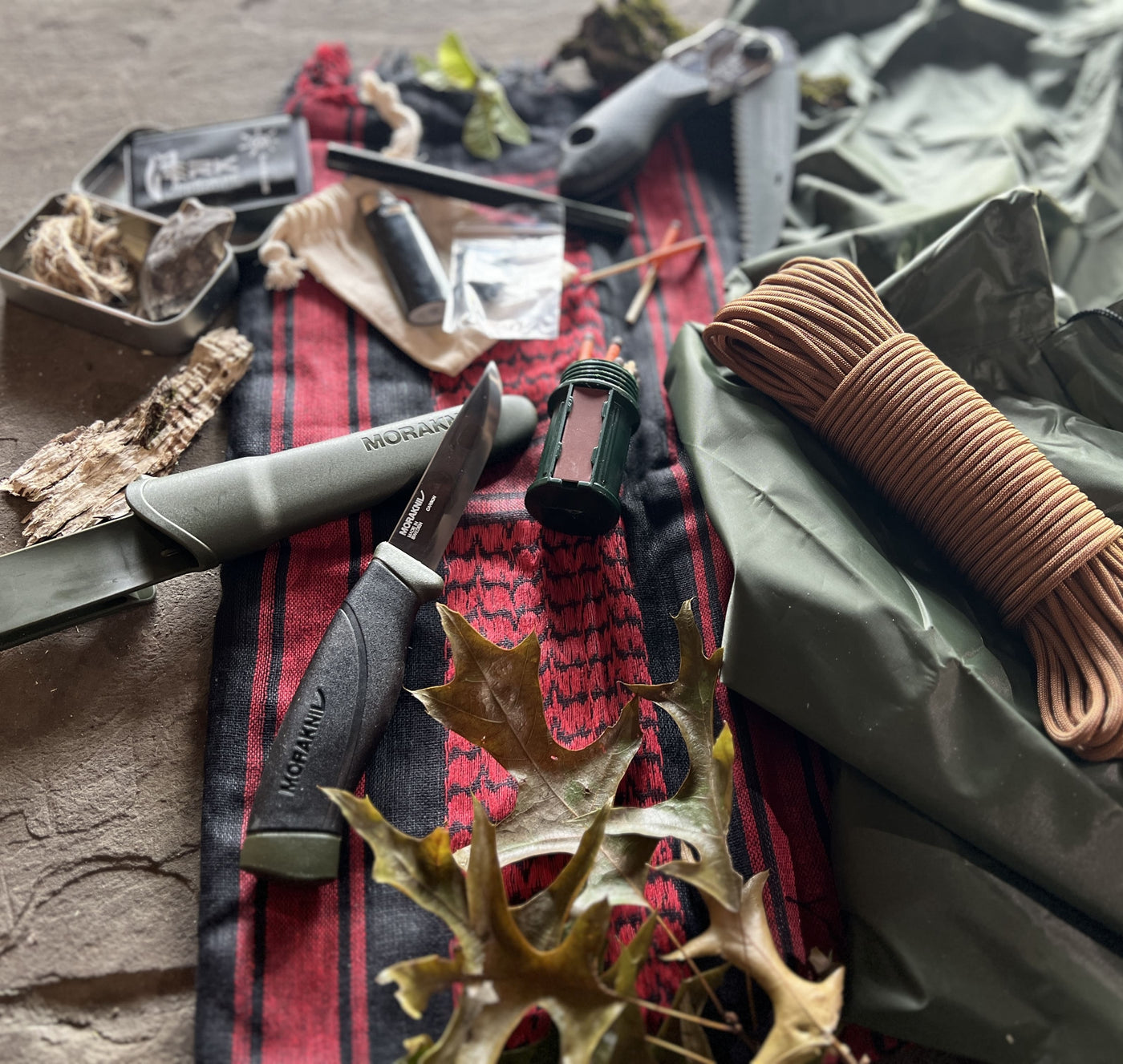The image depicts a diverse array of camping and survival gear, meticulously laid out on the ground. Central to the scene is a rumpled, partially unfolded tarp or possibly a deflated tent, covered in a scattering of dried leaves which lends a rustic tone to the setup. Spread across the surface is a compact fire starting kit that includes a lighter, matches, and a small pouch, possibly containing tinder materials. Occupying the right side of the image is a durable, rolled up bundle of paracord. 

In the middle of the frame, there is a collection of knives. Most prominently, there is a Morakniv pocket knife with its sheath extending to the left, alongside another fixed-blade knife with a short, robust blade. Near these tools, there is a small container, potentially a waterproof matchbox, indicative of the rugged environment and preparedness of the scene.

Adding a touch of color, there is a distinctive red and black cloth beneath the larger items, possibly a shemagh or a similar patterned accessory, enhancing the utility and survival aesthetic. This cloth is partially obscured by the various tools and equipment, including a gunmetal-colored tin box reminiscent of an Altoids container, which might be holding smaller survival essentials. In the background, a small retractable knife is visible, complementing the array of practical gear.

Overall, the assortment includes not just knives and fire-starting tools, but also elements suggesting a thorough preparation for outdoor living, implying that the owner is well-equipped for wilderness survival or an extended camping expedition.